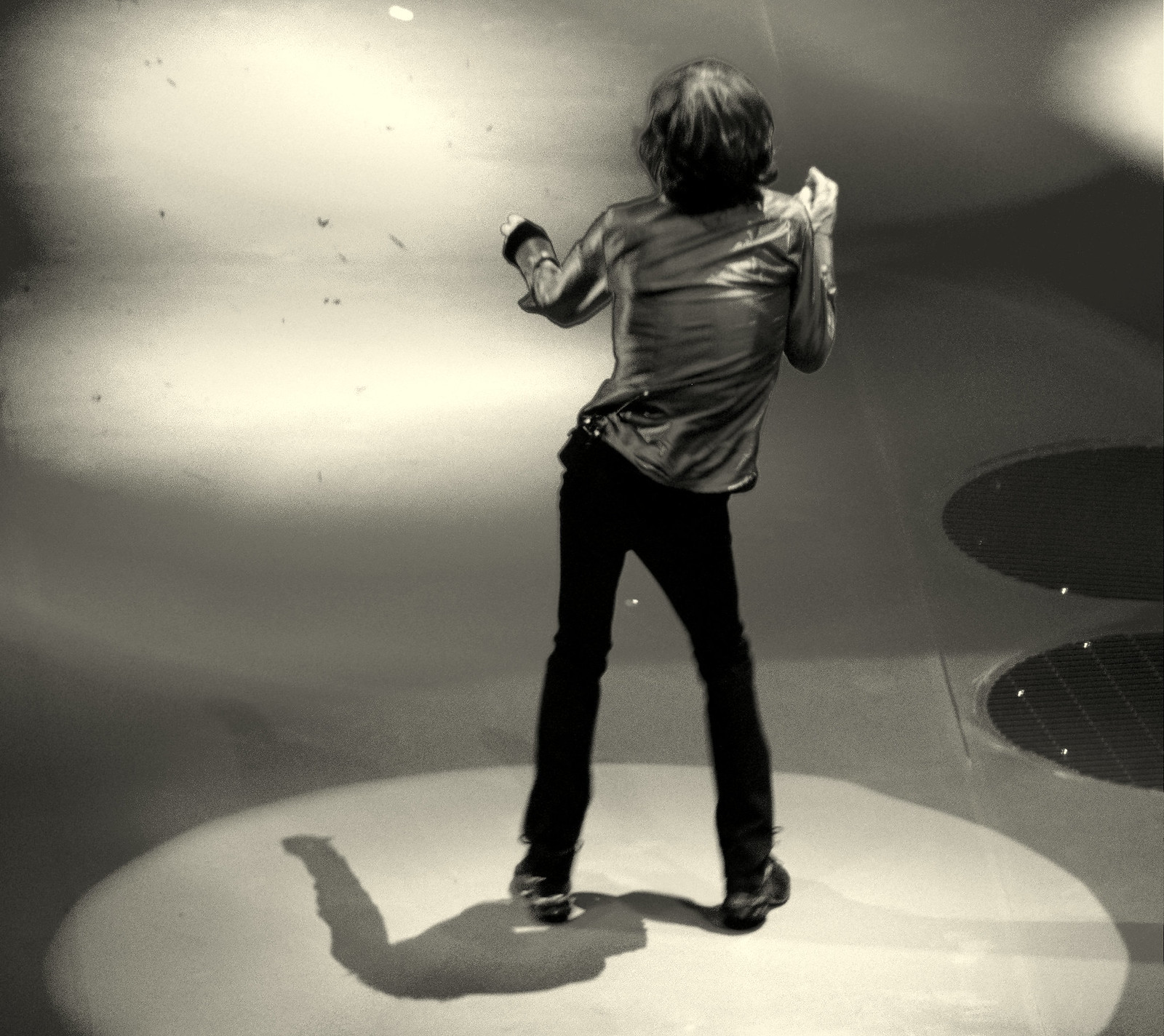A man, reminiscent of Mick Jagger, is dancing energetically on a stage, facing away from the camera. He is wearing a reflective jacket, dark pants, and dark shoes, with a hairstyle that strongly evokes the iconic rock star. A bright spotlight shines on him from the right-hand side, creating dramatic lighting and casting multiple shadows. This central spotlight is joined by at least two other light sources, enhancing the stage's vibrant atmosphere. The scene appears to be set in a discotheque or a similar lively venue. The entire image is in black and white, giving it a vintage feel. Despite the energetic dance movements, he is the sole performer visible on the stage.